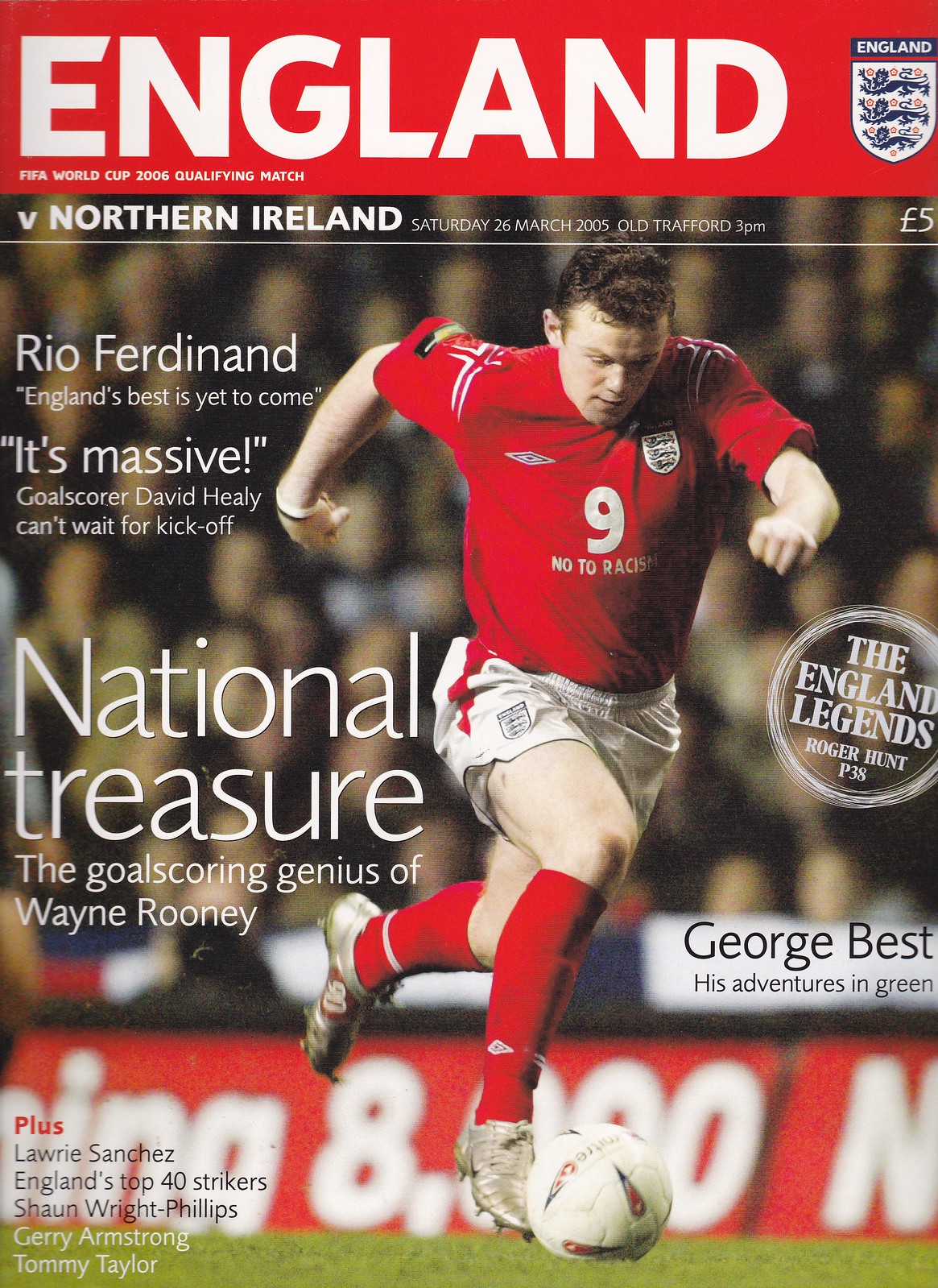The magazine cover prominently features an action shot of a football player in a red jersey with white shorts, red socks, and white cleats, running and kicking a soccer ball. The background reveals a stadium filled with spectators. Across the top of the cover, a red strip with white font reads "England" and "FIFA World Cup 2006 Qualifying Match." An England crest is located in the top right corner, along with the price, "5 pounds." Below, text details the event: "Northern Ireland, Saturday, 26 March 2005, Old Trafford, 3 p.m." The magazine highlights various articles, such as "Rio Ferdinand: England's Best is Yet to Come," "It's Massive: Goal Scorer David Healy Can't Wait for Kickoff," "National Treasure: The Goal-Scoring Genius of Wayne Rooney," "The England Legends: Roger Hunt (Page 38)," and "George Best: His Adventures in Green." Additional features at the bottom left include, "Plus: Laurie Sanchez, England's Top 40 Strikers, Sean Wright-Phillips, Jerry Armstrong, and Tommy Taylor."